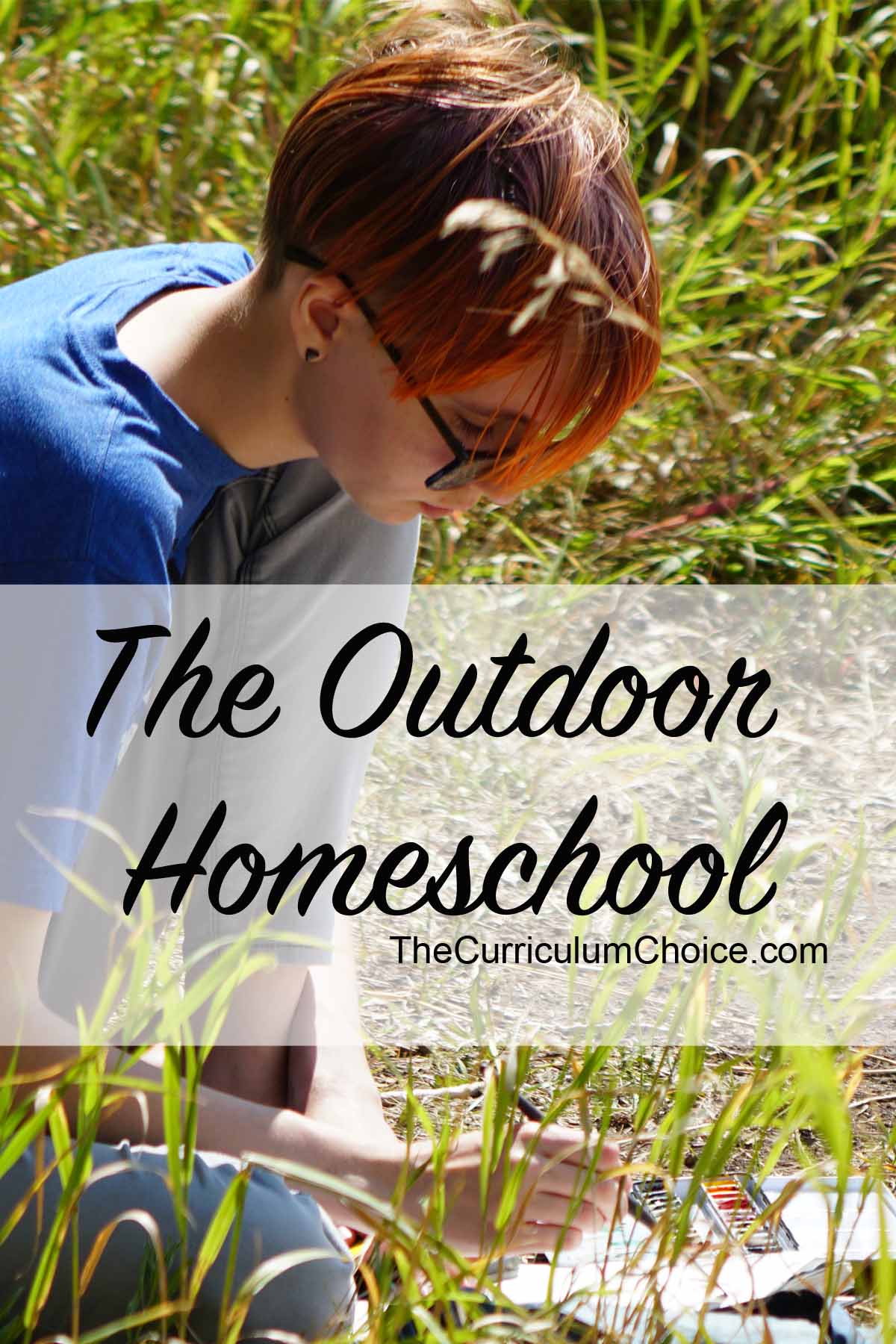This color photograph, oriented in portrait mode, serves as an advertisement for The Outdoor Homeschool and prominently features a slightly translucent white banner across the lower portion. In elegant black cursive script, the banner displays “The Outdoor Homeschool” with “thecurriculumchoice.com” printed in a smaller black font below. Depicted in the background is a young individual with red hair styled in bangs and short behind the neck, wearing dark-framed glasses, a blue t-shirt, and blue jeans. The person is kneeling on the ground amidst tall green and yellow grass, engaging in a watercolor painting session. They are seated with one knee up under their chest and the other leg folded underneath. The right hand is holding a paintbrush, dipping it into a tin of watercolor paints resting on a partially obscured white sheet of paper. Scattered around them are hints of dirt and dry leaves, enhancing the outdoor setting. The photograph is a representation of realism combined with graphic design elements, capturing a serene moment of creative learning in a natural environment.